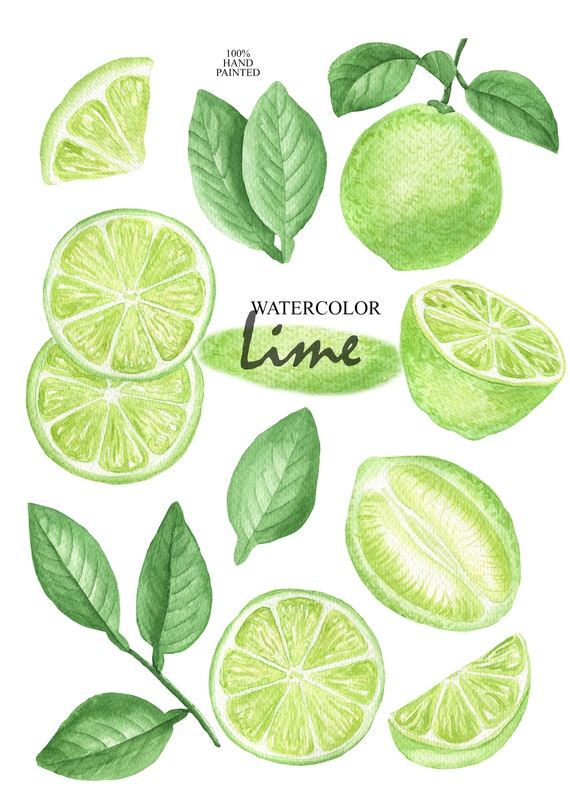The image is a detailed watercolor poster featuring various depictions of limes. At the top of the poster, the words "100% hand-painted" are prominently displayed, indicating the artisanal nature of the artwork. The center of the poster showcases the word "lime" written elegantly in cursive over a lime green oval, with the word "watercolor" printed above it.

Throughout the predominantly white background, the poster artistically illustrates different forms of limes and lime leaves. In the top left corner, there is a lime slice next to some lime leaves. Moving to the top right, there is a whole lime complete with its stem and leaves. The middle of the poster features two lime wheels on the left, with a half lime on the right. In the bottom section, a round slice of lime occupies the middle, flanked by a whole lime with two wedges taken out on the right, and another branch with leaves on the left. The various shades of green, from the darker leaves to the lighter limes, add depth and realism to the hand-painted artwork, capturing the vibrant essence of the fruit.